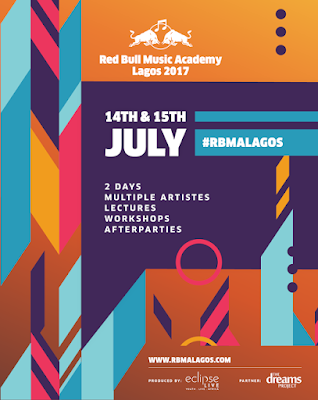The image depicts a vibrant and eye-catching poster for the Red Bull Music Academy in Lagos, 2017. The design features a harmonious blend of muted bright colors including oranges, purples, light blue, dark blue, dark pink, and a golden yellow. The left side is adorned with intricate patterns that add a unique artistic touch.

Prominently displayed are the event dates, "14th and 15th of July," along with the hashtag "#RBMALAGOS." The text emphasizes the numerous activities planned for the event, stating "Two days, multiple artists, lectures, workshops, after parties." 

Towards the bottom, the words "Eclipse" and "Dreams Project" are visible, hinting at some of the featured segments or themes. The overall design exudes a lively and inviting atmosphere, making it clear that this event was a must-attend for music enthusiasts in 2017.